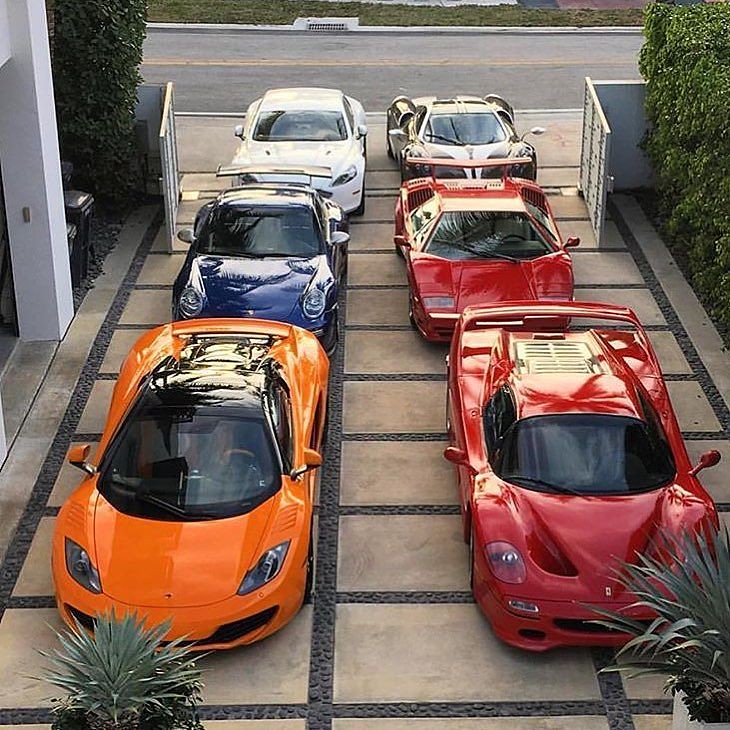The image depicts six high-end sports cars arranged in two parallel rows of three, parked in an elaborate driveway with a grid-like stone paneling design. Starting from the top left in the first row, the cars are: a white sports car, a navy blue Porsche, and an orange sports car with a black roof and tail fin. In the second row starting at the top, there is a sports car that appears to be either black or brown with white detailing, followed by two red cars, one of which has tinted windows. The setting is an upscale property with an open gate allowing access from the street, and there are plants accenting the corners of the photograph, adding to the image's luxurious ambiance. Based on the visible badges, the cars are potentially prestigious brands like Ferrari or Lotus, highlighting their opulence and exclusivity.